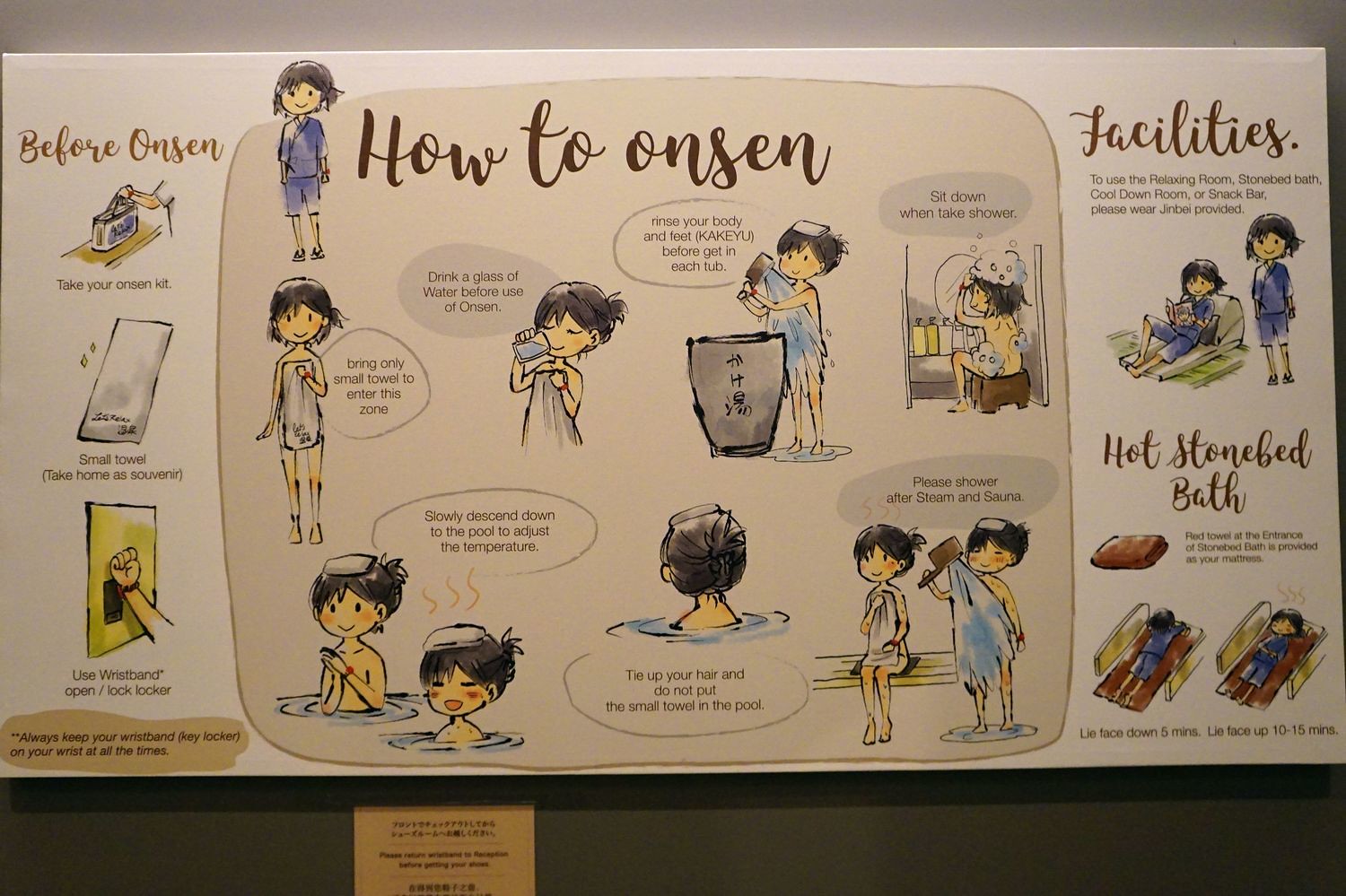The image is a detailed, color photograph of a poster inside an interior facility, presented in landscape orientation. The poster provides an elaborate guide on the onsen experience, featuring a white background with black type and vibrant color illustrations. In the center, bold script text reads "How to Onsen." To the left, under the heading "Before Onsen," three illustrations depict preparations such as taking out an onsen kit, using a wristband, and unlocking a locker. A stick figure character with shoulder-length dark hair is depicted smiling, dressed in a blue top and shorts, and is shown showering with blue water on her body. The onsen instructions emphasize bringing only a small towel, slowly adjusting to the pool temperature, staying hydrated, and rinsing thoroughly before entering each tub. It also advises tying up hair and refraining from putting the small towel in the pool. The right side of the poster, under "Facilities," lists amenities like a relaxing room, stone bed bath, and a snack bar, where participants utilize a provided Jinbei. Specific instructions for the hot stone bed bath include using a red towel as a mattress and timing positions for lying face down and face up. Through rich, representative illustrations and detailed text, the poster comprehensively guides visitors on enjoying the onsen experience.